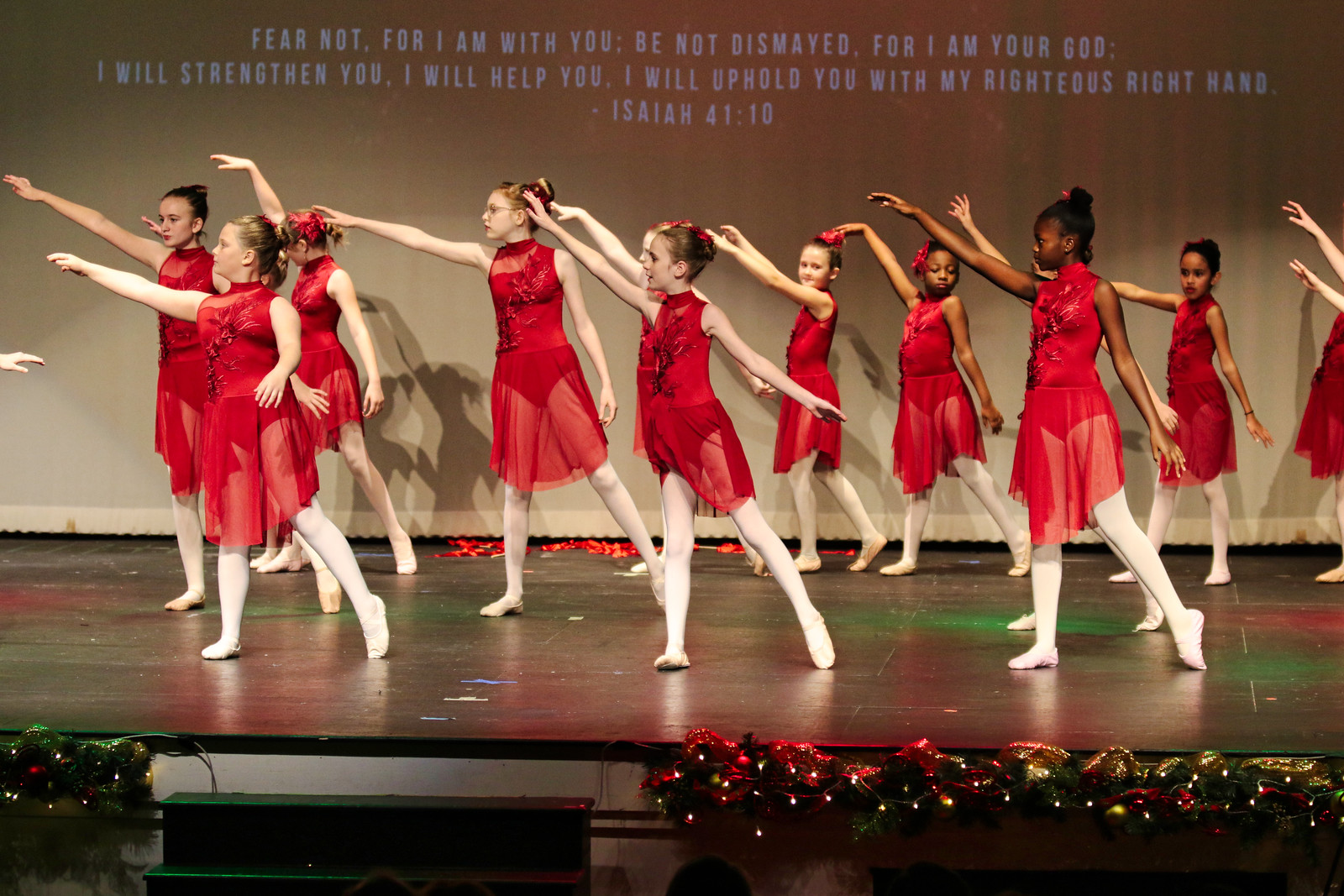This photo captures a group of middle school-aged ballet dancers performing at a dance recital. The dancers are dressed in red, sleeveless leotards adorned with a sheer skirt and a floral applique on the front. Complementing their outfits, they wear white tights, ballet slippers, and red ribbons in their hair, with their hair styled in buns. The girls are all striking a coordinated pose, stretching their right arms forward and extending their left legs backward. They are positioned on a stage decorated with Christmas plants and illuminated by red and green lights. In the background, white text projected onto draped curtains features the biblical verse Isaiah 41:10 in blue writing: "Fear not, for I am with you; Be not dismayed, for I am your God. I will strengthen you; I will help you; I will uphold you with my righteous right hand."